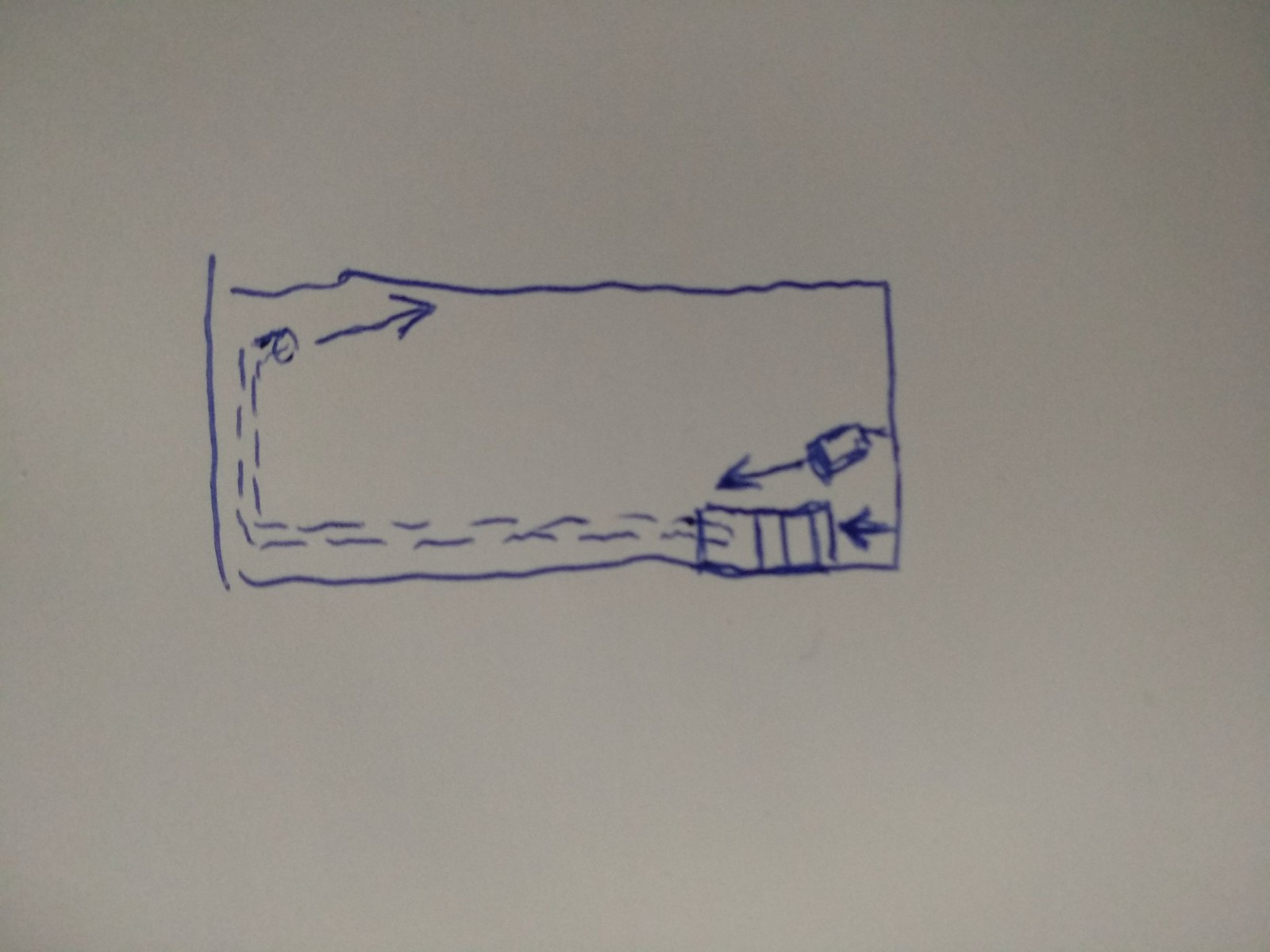The image is primarily white, featuring a roughly sketched blue rectangle at its center. 

- In the bottom right corner of the blue rectangle, there is a hand-drawn cylinder with an arrow extending outwards.
- Below this cylinder, an arrow points towards another small rectangle filled with vertical stripes.
- Emerging from the striped rectangle, there are double-layered dashed lines that stretch horizontally from right to left. Upon reaching the left side, the dashed lines make a turn and extend vertically up the side of the rectangle.
- Near the top of these dashed lines, there is another cylindrical shape. Outside this shape, an arrow points back towards the right-hand side.
- The top line of the entire blue rectangle does not completely connect at the upper left corner.

The image seems to depict a sequence or flow of processes with directional arrows and connecting lines, though the specific details and purpose are abstract in nature.